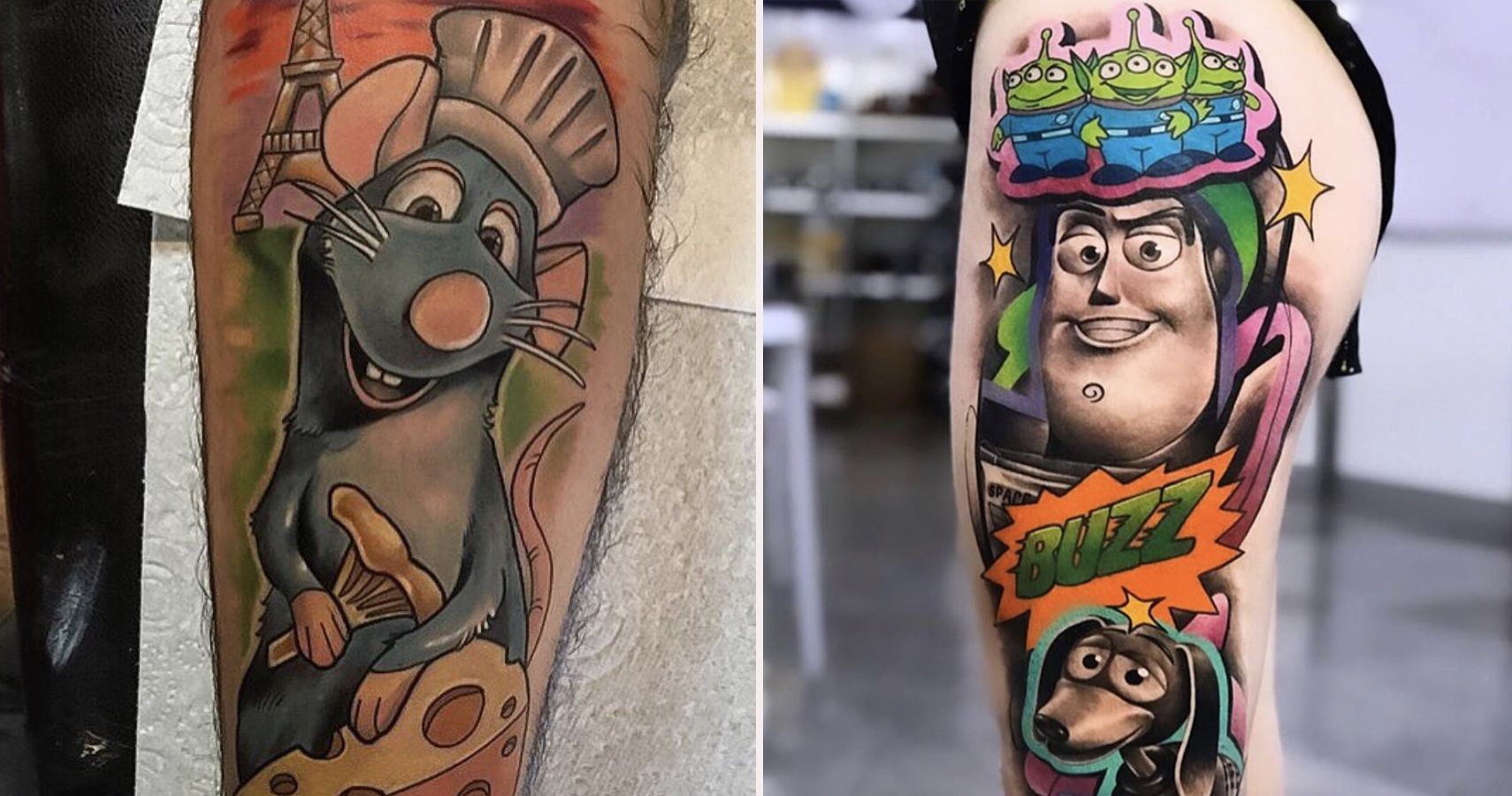This image showcases two detailed and vibrant Disney Pixar-themed tattoos side by side. The left photograph displays a fully colored, realistic tattoo on the underside of an arm. It features Remy, the endearing blue rat from *Ratatouille*, wearing his chef's hat. Remy is depicted holding a piece of cauliflower in one hand and a piece of cheese in the other, with the Eiffel Tower prominently in the background and accents of a green and red sky. The right photograph captures a tattoo on what appears to be the upper thigh area. This eye-catching mural includes Buzz Lightyear from *Toy Story*, framed by smiling three-eyed green aliens atop his helmet. Below Buzz’s face is his name ("BUZZ") written in green letters, and beneath that is Slinky Dog, surrounded by a few stars. In the background of the right photograph, a tattoo shop can be faintly seen. Both tattoos are richly colored and intricately detailed, celebrating beloved Pixar characters with a vibrant and playful aesthetic.